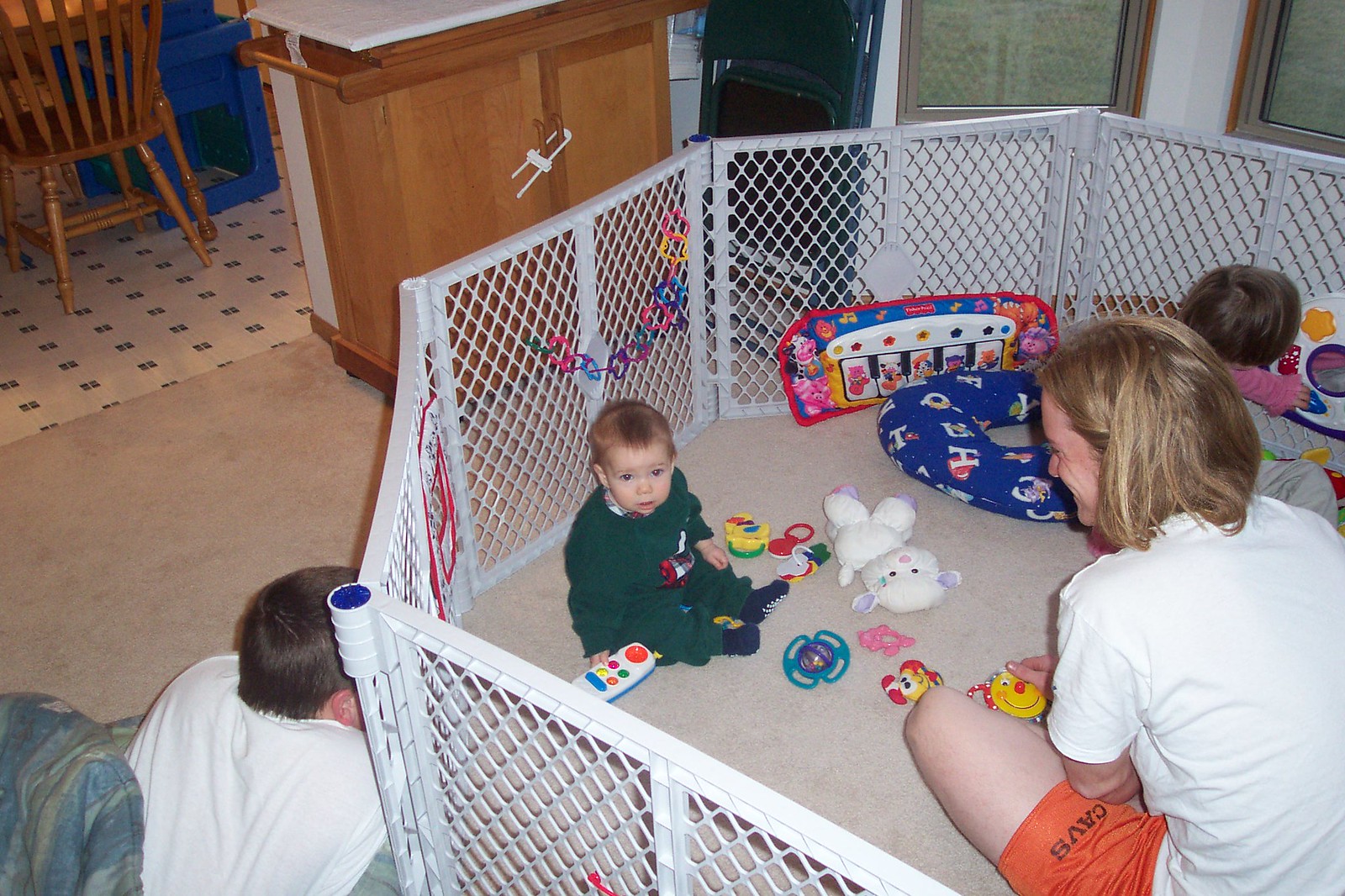In this photograph, an old-style image captured with an older camera, we see a family scene focused around a white, octagon-shaped playpen made out of interconnected baby gates with diamond-shaped spaces. Inside the playpen, a mother with shoulder-length blonde hair, wearing a white short-sleeve shirt and orange athletic shorts, sits smiling at two children. A baby boy wearing a dark green outfit sits on the ground looking at the camera with a slightly puzzled expression, surrounded by various toys including a stuffed bunny, a toddler's keyboard, a toy phone, a teddy bear, a white stuffed cat, and spinners. To the top right within the playpen, a baby girl dressed in pink plays with another toy, her back facing the camera. Just outside the playpen on the left, a man with short brown hair wearing a white t-shirt lies on the floor, watching the children play.